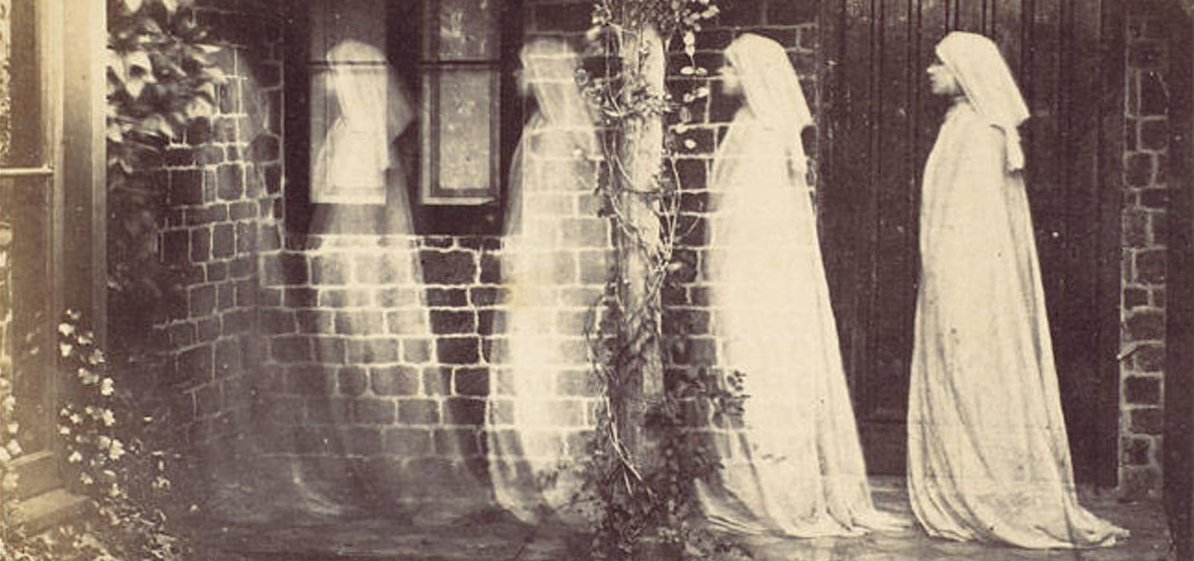The black-and-white photograph, reminiscent of an old-time image, exudes an artistic feel. The scene captures the exterior of a brick building, characterized by a brown door on the left and a two-paned window on the right. A perpendicular brick wall with additional windows extends beyond the main focus. Intricate details include greenery and ivy climbing the side of a window and a column adorned with flowers nestled between the door and window. Central to the image is a series of a single woman, likely a nun, clad in a long white gown and white habit, her face visible only in the first instance. The woman appears multiple times across the frame, starting on the left in solid form and gradually becoming more ghostly and translucent as she moves towards the right. This fading effect continues over five iterations until she nearly disappears into the building wall, accentuating a spectral transformation. The ethereal progression of her figure adds a haunting yet captivating element to the historical aesthetic.